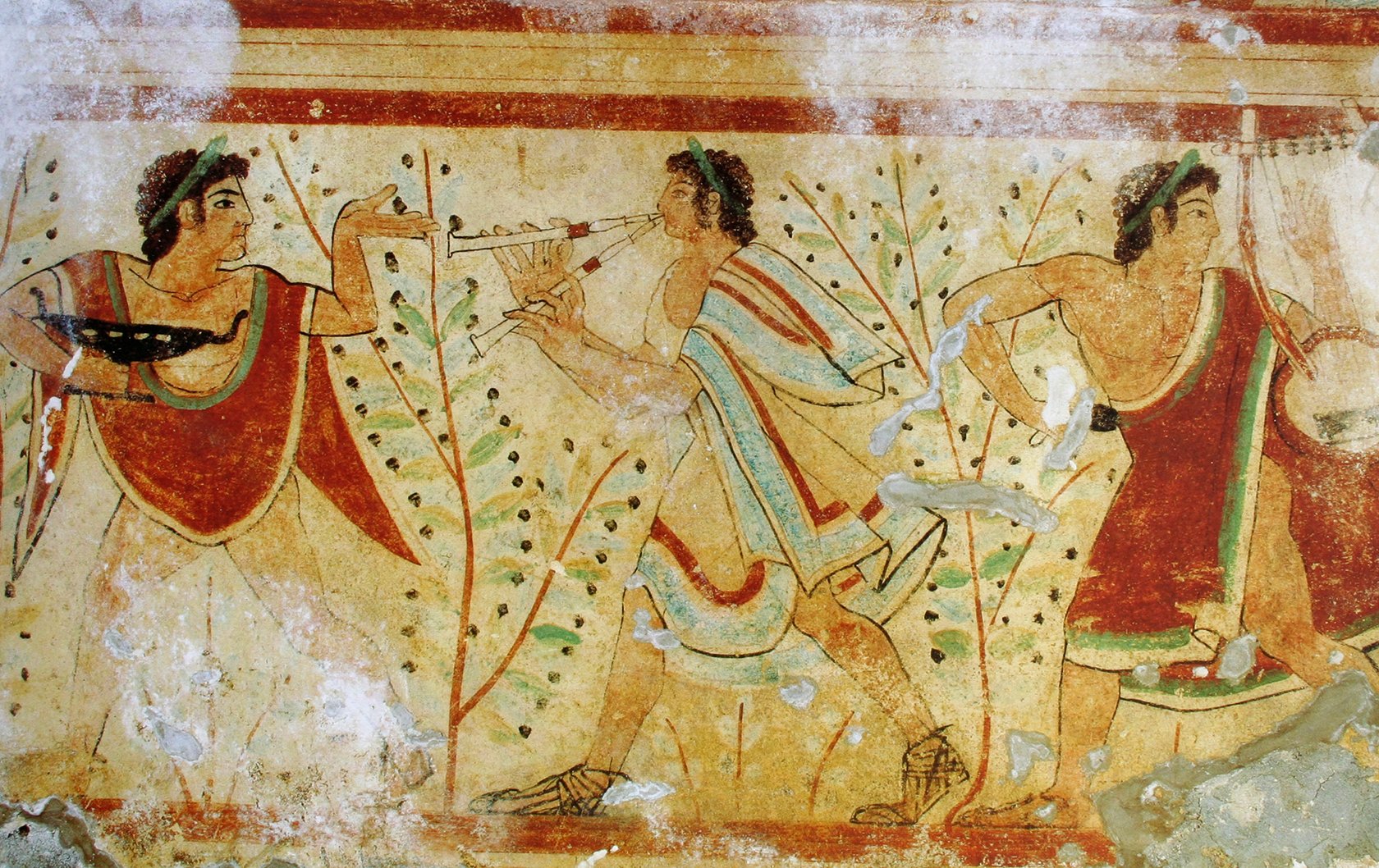This photograph captures a weathered, ancient painting on a stone wall, depicting three figures in a simplistic yet evocative style. The first figure, positioned to the right, raises his left hand in an offering gesture, while his right hand clutches a black vessel. The central figure faces left, holding two flutes adorned with white and red stripes, his movement suggested by his forward posture. He wears flowing white robes highlighted with blue and red stripes. The final figure, garbed in a red robe with green and white striped edges, gazes rightward, absorbed in playing a harp. The backdrop is a stark white, accentuated by at least two plants bearing green leaves and dark fruits. A red border frames the entire scene, emphasizing its antiquity and artistic significance.